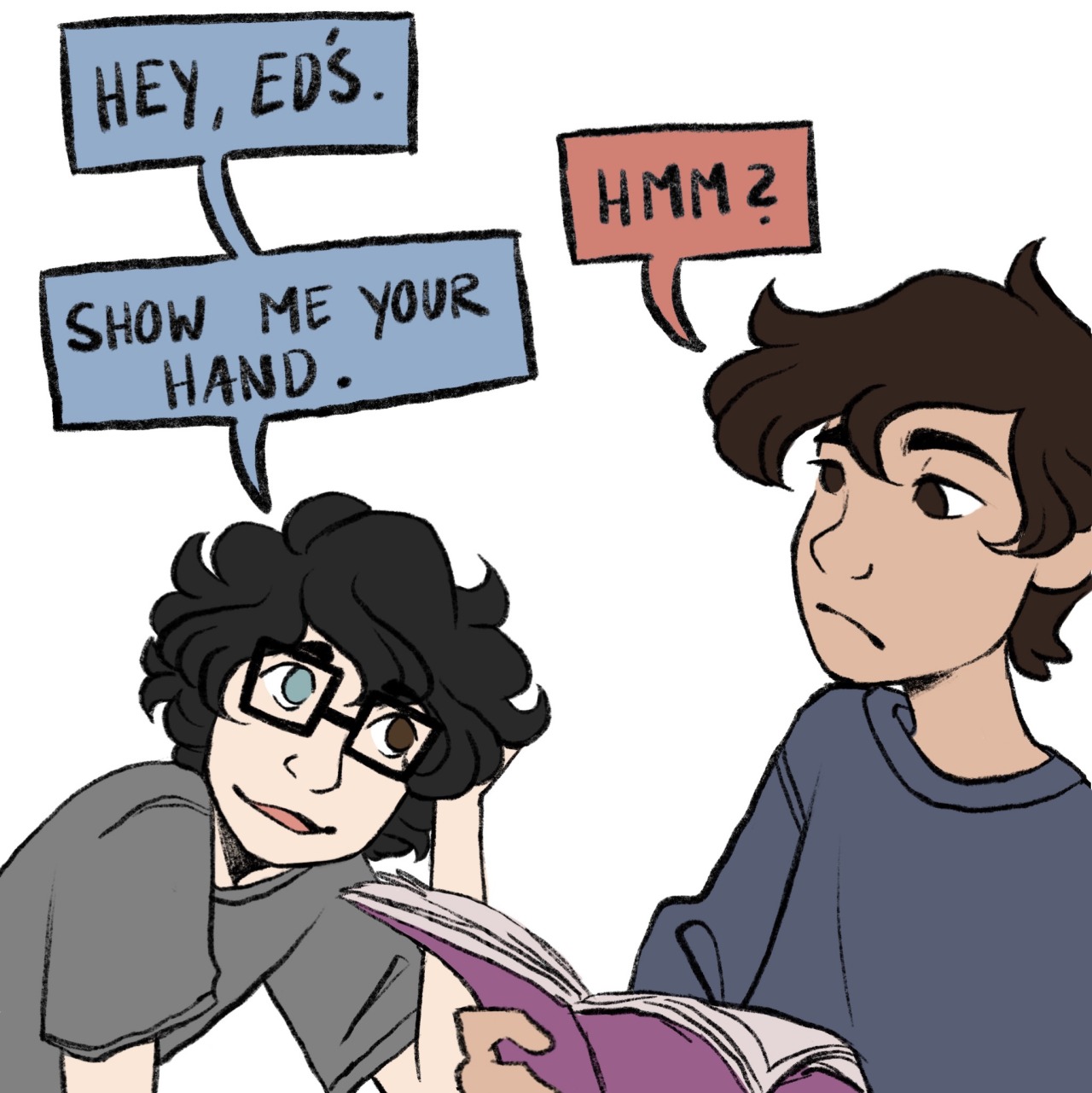In this hand-drawn, slightly cartoonish comic panel, two young men are depicted. On the left, a character with medium-length, bushy black hair and square-framed glasses stands out. His heterochromatic eyes—one green and one brown—add a unique touch to his appearance. He has very pale skin and wears a gray shirt. The young man on the right has brown hair and tan skin. He gazes attentively with his brown eyes, dressed in a bluish shirt, while holding an open purple book. The scene includes two text bubbles. The dialogue begins with the left-hand character saying, "Hey Eds," followed by the right-hand character responding with, "Hmm." The left-hand character then adds, "Show me your hand."